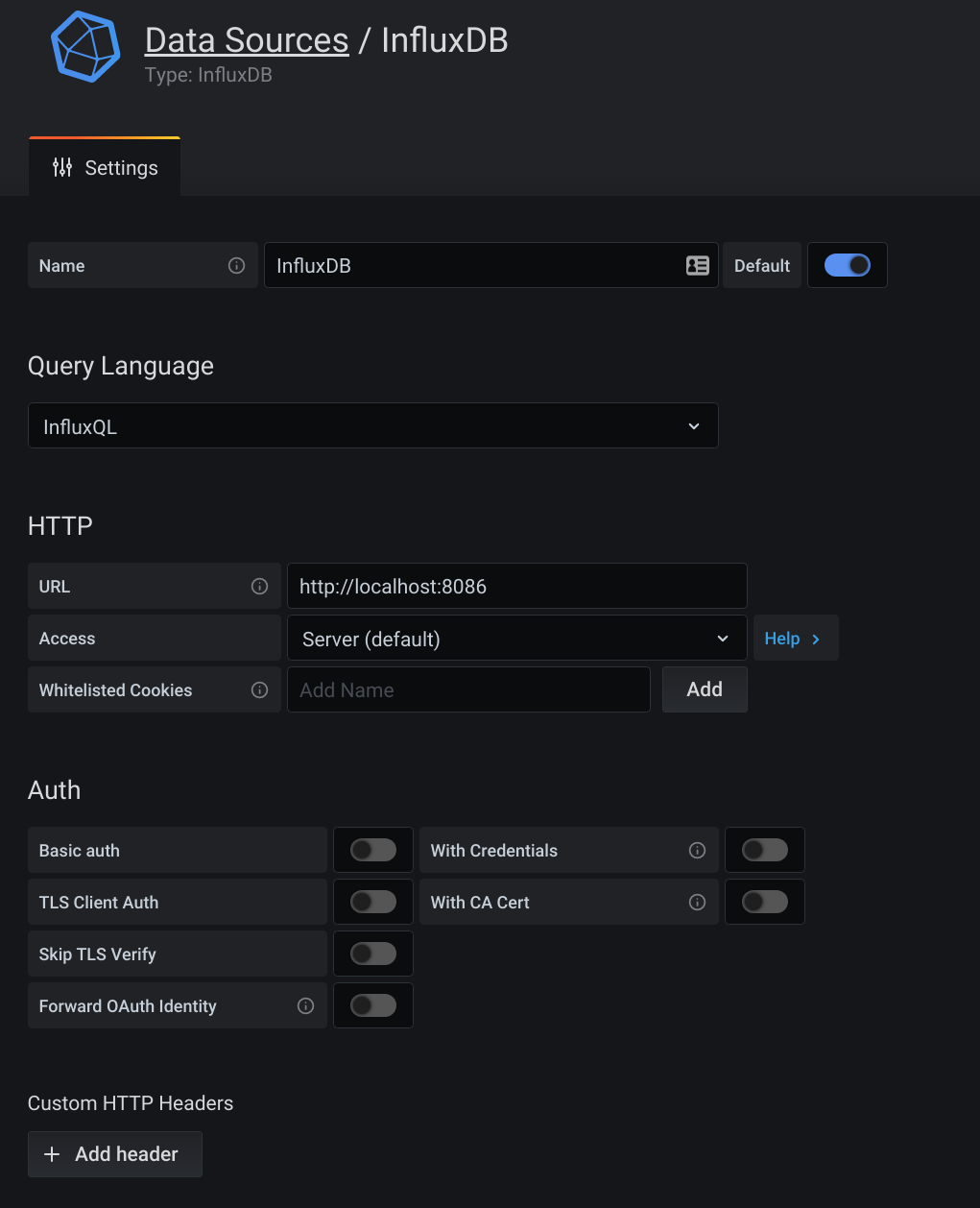The image showcases a detailed configuration screen for a data source setup in a software interface. At the top left, there is a blue geometric icon. To its right, in white text, it reads "Data Sources," which is underlined, followed by "InfluxDB" without any underlining. The letters "I," "D," and "B" in "InfluxDB" are capitalized.

Beneath this header, in a smaller light gray font, the text reads "Type InfluxDB." Below, on the left side, there is a "Settings" label with an orange bar above it and a settings icon to the left. 

Underneath the settings label, the name "InfluxDB" is shown as the chosen data source name. The option "Default" is toggled on, indicated by a blue button. Further down, there is a "Query Language" dropdown menu in white text, with "InfluxQL" selected as the option.

Additionally, in bold white text, there is an "HTTP" label directly under which a URL setting is displayed: "HTTP" is selected, and the text box beside it contains "http://localhost:8086." The "Access" dropdown menu is set to "Server Default."

To the right, there is a "Help" button. Beneath this section is a label for "Whitelisted Cookies" with a text box for adding names, which currently has no entry. The box prompts the user to "Add Name."

This thoroughly describes the structure and elements of the configuration screen, highlighting all the selected and default settings included.